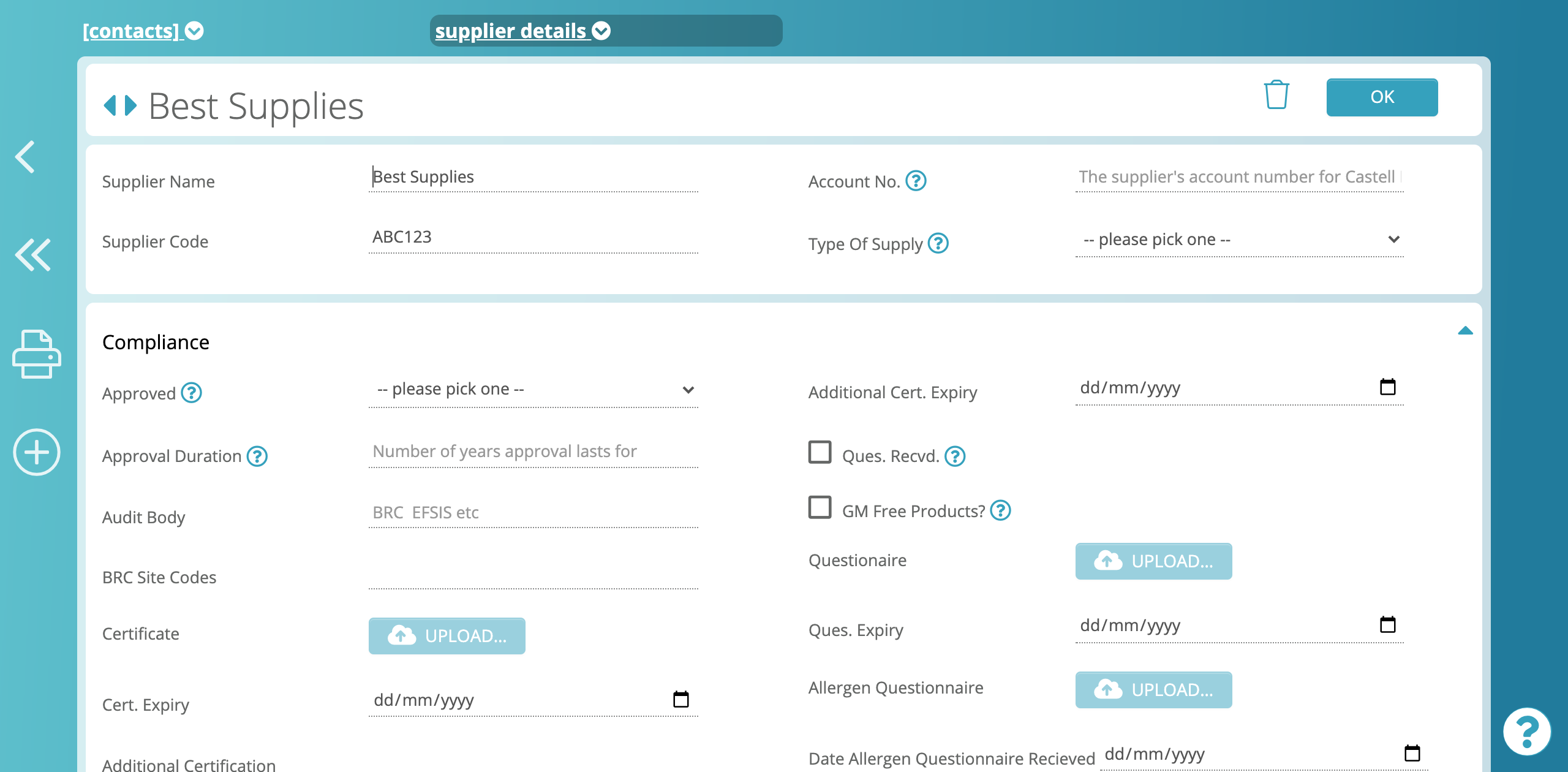This image showcases a computer screen displaying contact information within a user interface. The screen background is a calming light blue hue. At the top, there's a section labeled "Contacts" with a drop-down menu beside it, followed by another labeled "Supplier Details" in a darker blue bar, also featuring a drop-down menu.

On the right side, a white circle with a question mark is hovering in the corner, possibly for help or additional information. On the left side, a vertical toolbar includes navigational options—an arrow pointing left, double arrows pointing left for quicker navigation, a print symbol, and a circle with a plus sign for adding new entries.

The main information area has a white background. The interface prominently shows "Best Supplies" at the top with a trash can icon to delete the entry and an "OK" button to save changes. Below, detailed information about the supplier is listed:
- **Supplier Name:** Best Supplies
- **Supplier Code:** ABC123
- **Account Number:** (empty field for input)
- **Type of Supply:** (dropdown menu with the text "Please pick one")
- **Compliance Approved:** (dropdown menu with the text "Please pick one")
- **Additional Cart Expiry:** (field for date input or a clickable link to access a calendar)

Further down, there are sections for:
- **Approval Duration:** Indicating the number of years for which the approval is valid.
- **Audit Body:** Listing options like BRC, EPSIS, etc.
- **BRC Site Codes:** (field for input)
- **Certificate:** (option to upload a picture)
- **Questionnaire:** Including fields for question expiry, allergen questionnaire, and certification expiry.
- **Additional Certification:** (field for input)

The layout and options suggest a comprehensive and organized system for managing supplier information.